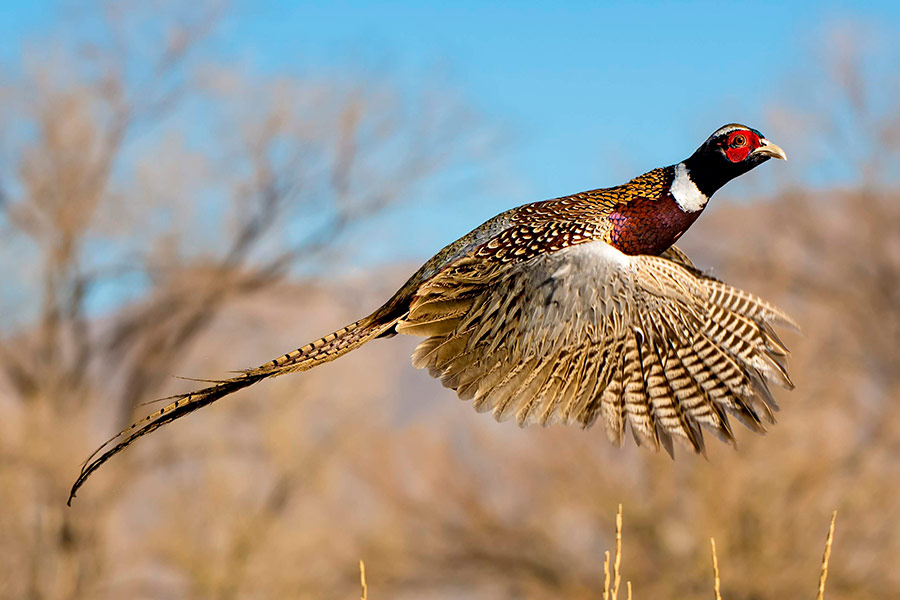In this outdoor image, the focus is on a magnificent bird, likely a pheasant or perhaps a sage hen, that has just taken flight. The bird dominates the scene, with its black head and a distinct white ring encircling its neck. A splash of red around its eye and a striking yellow beak add vibrant details to its face. Its breast features maroon tones, seamlessly transitioning to tan feathers on its body and brown wings adorned with delicate wingtips.

The pheasant's tail extends impressively, almost matching the length of its body. Behind the bird, the background is artistically blurred, showcasing a clear blue sky devoid of clouds. Bare tree branches and the subtle gray-tan hues of distant hills and mountains set a serene backdrop. Closer to the camera, a few stems of foliage are visible, providing a natural frame to this dynamic avian subject. The overall scene exudes a sense of wild beauty and peaceful coexistence with nature.